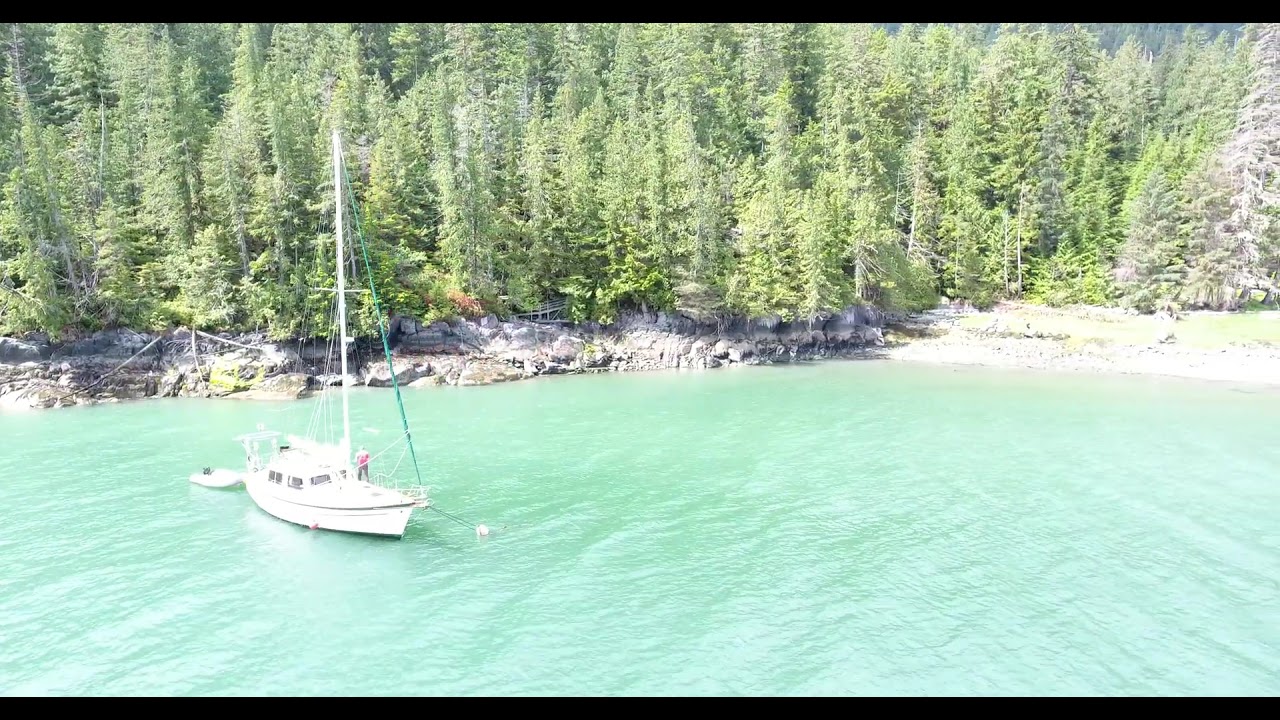In this brightly lit image, the sun bleaches the scene, causing a strong reflection off the white elements. Central to the image is a white, single-mast sailboat anchored on pristine, turquoise water that displays minimal ripples. The water is clear and clean, contributing to the serene atmosphere. Onboard the boat is a person in a red top and gray bottoms, standing near the masts. Attached to the back of the boat is a raft equipped with an outboard motor, and a line extends from the boat to its submerged anchor.

In the background, towering evergreen trees, resembling overgrown Christmas trees, rise above rocky white cliffs that are approximately 12 feet high. These rugged cliffs extend directly from the water's edge. A railed walkway or bridge is visible among the cliffs, adding a subtle human element to the natural surroundings.

To the right of the image, the shoreline varies between rocky terrain and a small open area with flat grass and a hint of sand, providing a minimal contrast to the otherwise densely forested shoreline. There are no docks or sandy beaches, reinforcing the untouched beauty of this lakeside or harbor scene.